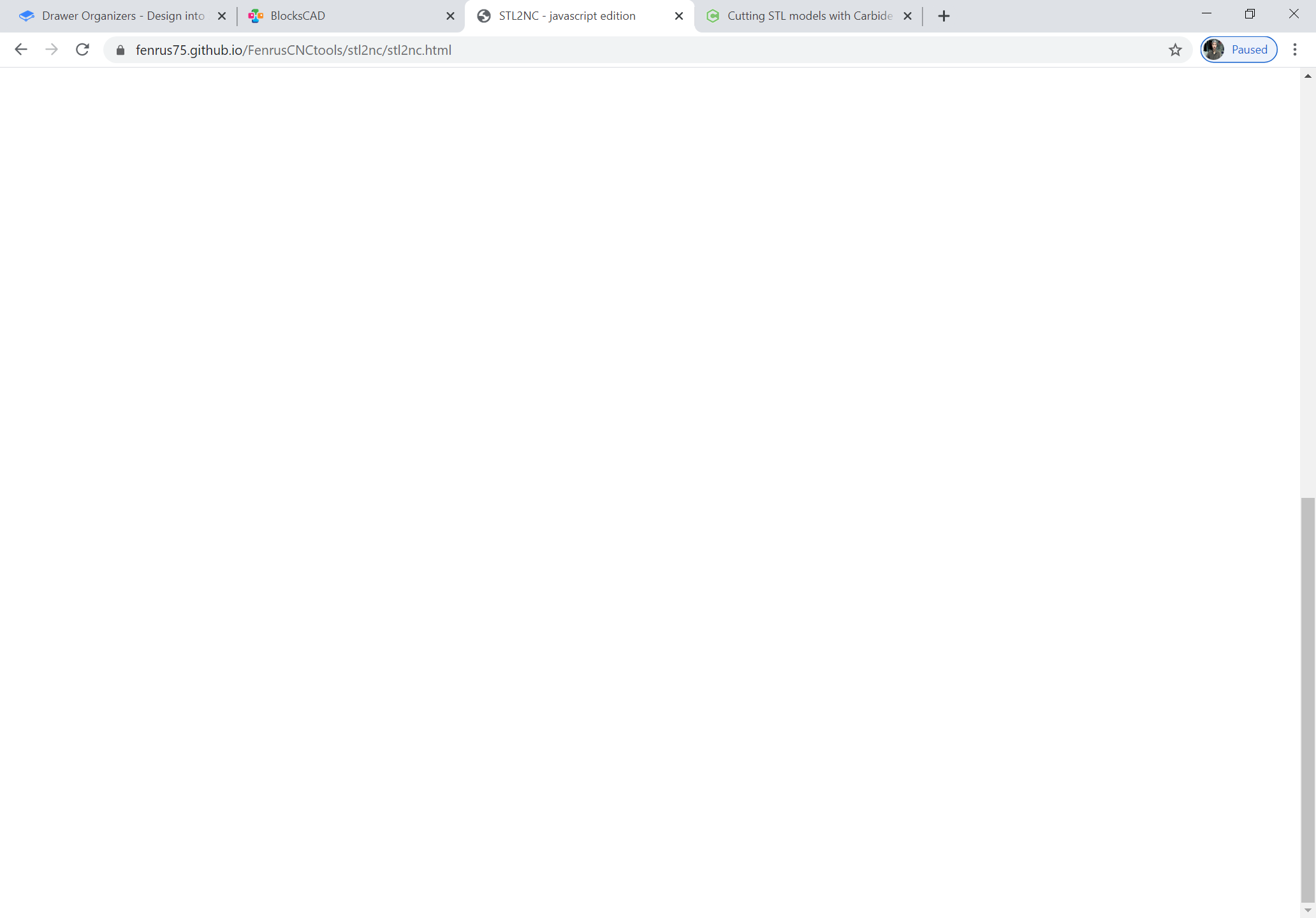This image depicts a completely blank white web page. At the very top, the browser tabs are visible, displaying the following titles from left to right: "Drawer, D-R-A-W-E-R Organizers, Dash Design Into..." with the latter part of the text truncated. This is followed by tabs labeled "BLOCKS CAD," "STL2NC JavaScript Edition," and "Cutting STL models with CARBIDE." The URL in the address bar reads "FENRUS75.GITHUB.IO/FENRUSCNCTOOLS/STL2NC/STL2NC.HTML". The central portion of the web page is entirely white and devoid of any content. There are no photographic, illustrative elements, people, or animals present in this image.